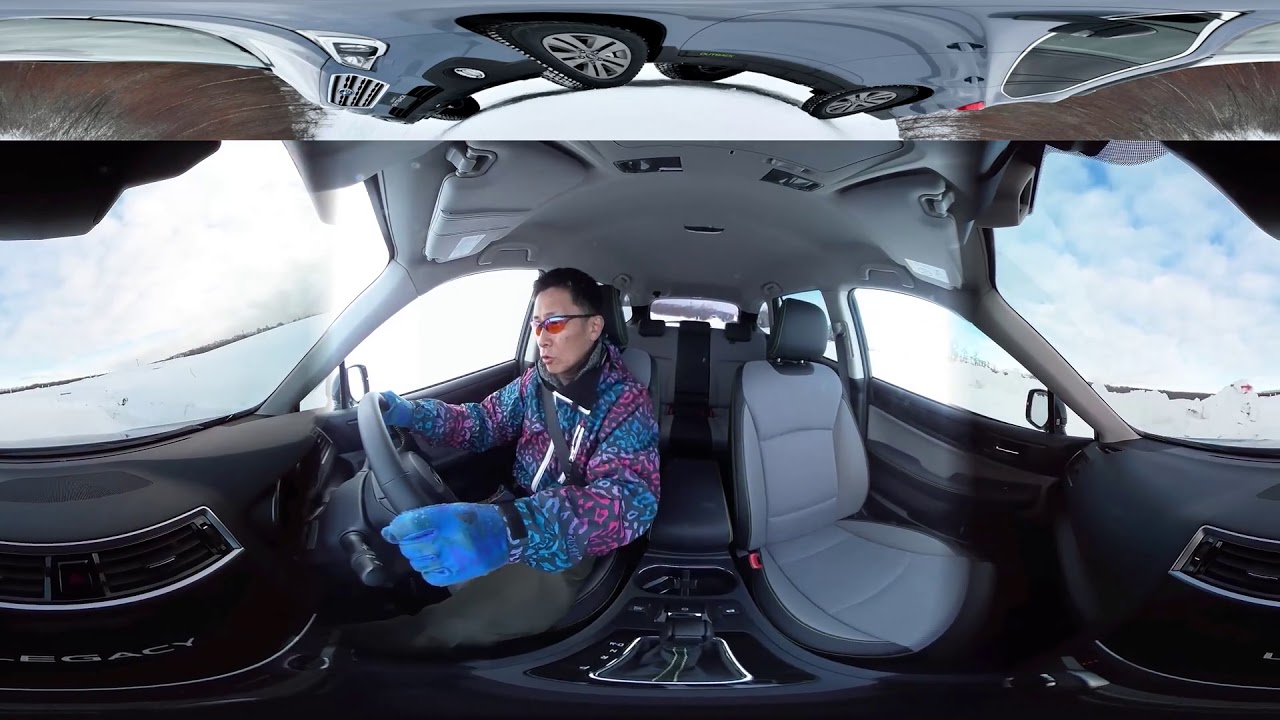The image is a composite with two distinct sections. The top part features the bottom view of a light blue vehicle equipped with studded tires driving over snow. The front grill is prominently visible, and the snowy landscape suggests a cold, winter environment. The bottom section provides an interior view of the car, revealing a clean cabin with grey and black accents, including grey seats and a central console with cup holders and a gear shift. In the driver's seat is an Asian man wearing a pink and green textured jacket, blue gloves, and orange sunglasses, with both hands on the steering wheel. Outside the car window, snow is visible along with a snowman. The entire image has a slightly stretched, curved appearance, with one seat facing right and the driver's seat facing left, enhancing the sense of motion and distortion in the photograph.